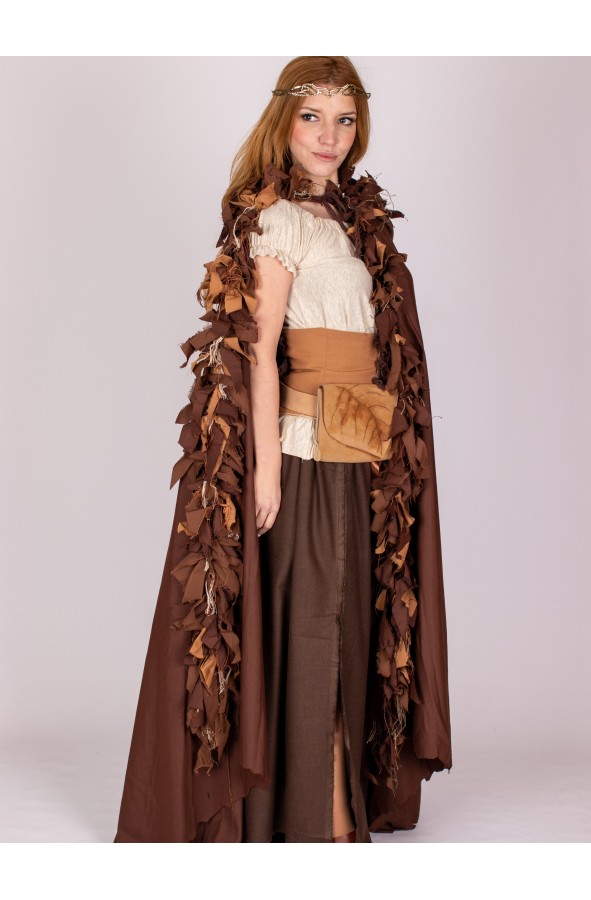In this image, we see a young woman standing against an off-white background, modeling a detailed medieval innkeeper or tavern keeper outfit. She is dressed in a large, long brown robe that reaches the ground, layered over an off-white peasant blouse with frilled details. This blouse is cinched at the waist with a light brown sash. Completing her ensemble, she wears a long brown skirt, which appears to have a slit on one side. Draped around her shoulders is a unique shawl, embellished with strips of brown fabric that mimic a scarf or garland of fabric leaves. 

Her long, reddish-brown hair cascades down her back, adorned with a metallic-looking thin headband, giving an impression of a subtle crown. With dark eyes, she gazes thoughtfully to the left-hand side. At her waist, there is a bag or pocket featuring a stencil of a leaf, adding to the authenticity of the medieval aesthetic. The overall look is intricate and reminiscent of a cosplay outfit, capturing the essence of a medieval female innkeeper with remarkable attention to detail.